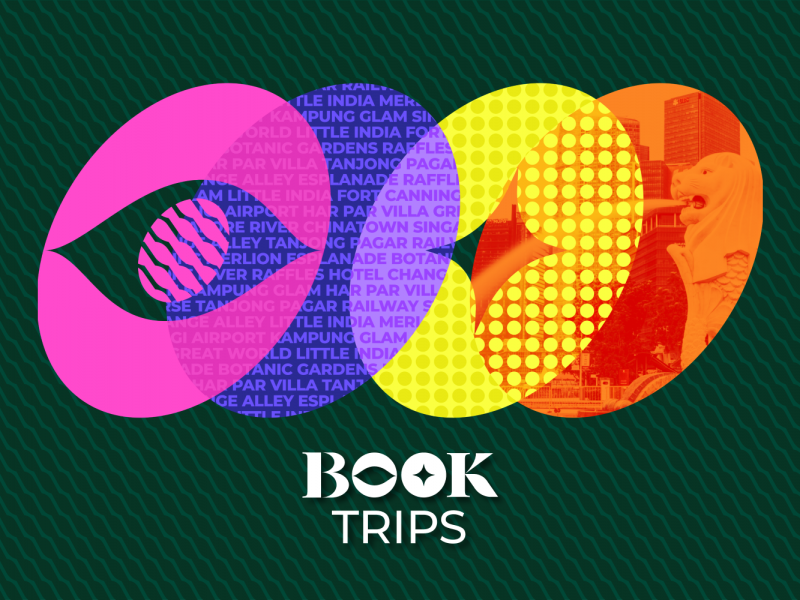The image depicts a vibrant, graphic design with a forest-green, textured background featuring wavy, horizontal lines. At the center are four overlapping, slanted ovals, each semi-transparent where they intersect. The oval on the far left is a purple eye shape with a detailed depiction of an eyeball, complete with a retina. Next to it is a blue oval filled with various repeating text, including words such as "India," "Parvia," "Chinatown," "Botanic Gardens," "Glam," "Little India," "Gardens," "Canning," "Change," and "Harparvilla." To the right of this is a yellow oval featuring a diamond shape, resembling a star or Christmas ornament. The fourth oval is orange and contains an image of a cityscape with a lion fountain. At the bottom of the image, in white text, is the phrase "Book Trips," with the two O's in "Book" stylized as the purple eye and the yellow star ovals.